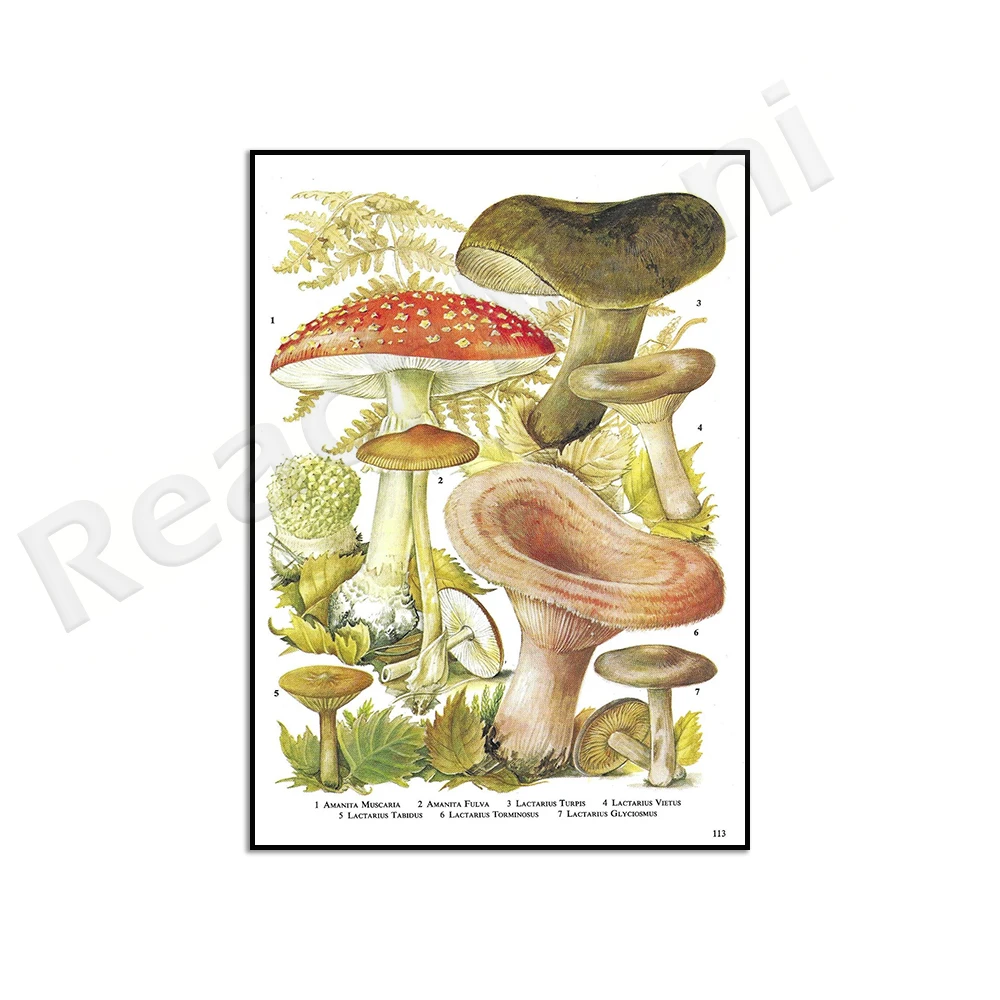In the illustration, a variety of whimsical mushrooms are arrayed against a white background, presented in intricate and detailed artwork reminiscent of botanical study guides. At the top right of the image, a distinctive black mushroom stretches upwards. Just below and to the left, a red-topped mushroom adorned with white spots stands out. Further down is a smaller brown mushroom with a notably long stem. Adjacent to it is another mushroom with a unique concave cap, which is somewhat unusual as it dips inward instead of curving downward. Nearby, there is a similar mushroom, slightly reddish with a central dip. Spread throughout the image are additional mushrooms including brown ones and a notable one on the left that resembles popcorn. Interspersed among the mushrooms are leaves in various shades of green, brown, and yellow, as well as some ferns in the background. Each mushroom is numbered, corresponding to names written in tiny print at the bottom of the image, likely their Latin taxonomy names, suggesting this piece could be from an educational textbook or a detailed field guide on fungi. The text at the bottom also seems to include the page number, which appears to be 113, indicating this could be a part of a larger compendium.